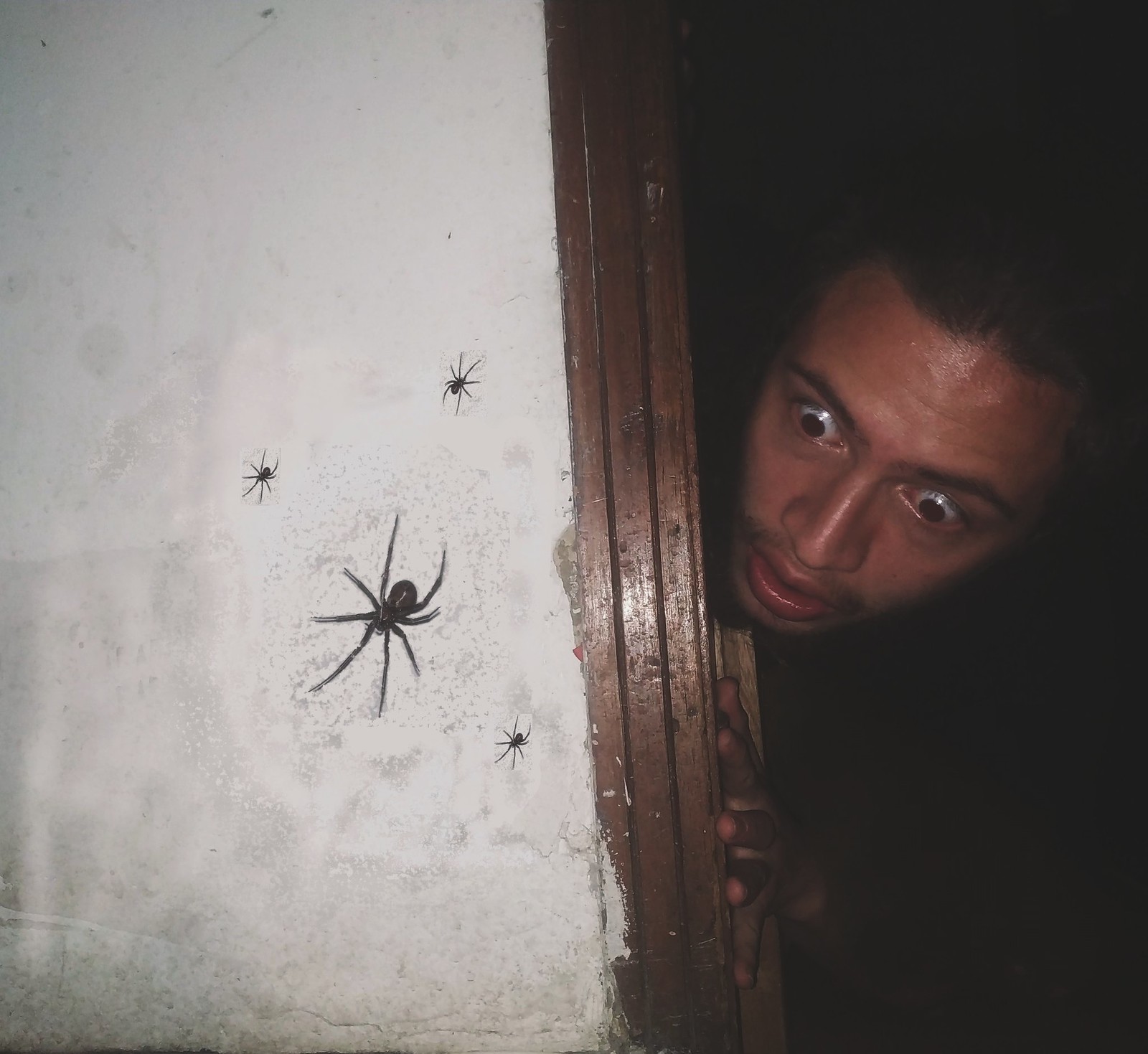In this photograph, a dark-skinned man with dark hair is peeking around the edge of a doorway, his hand gripping the frame. His eyes are wide open, clearly bugging out, and his expression is one of shock and stress. His slightly pink fingertips and reddish lips are noticeable. The scene behind him is very dark, perhaps indicating an unlit room. The wooden doorframe he clutches is dark brown, chipped, and shabby, contrasting sharply with the dingy, moldy, damaged white wall outside. On this white wall, to the left of the doorway, there is one large black spider, tarantula-like in its size with long legs, and three smaller baby spiders near it. The man appears extremely distressed by the sight of these spiders.